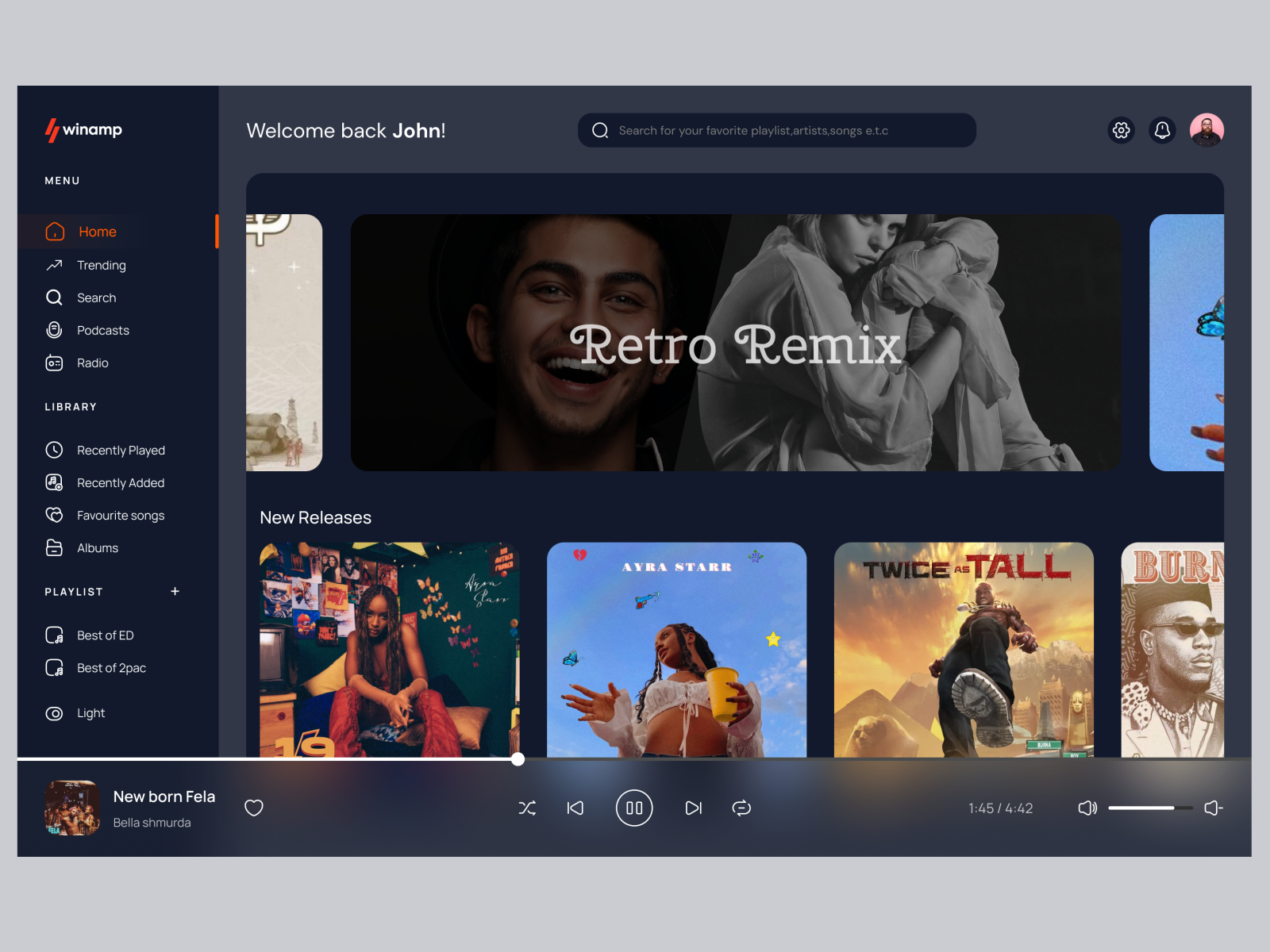This is a detailed screenshot of the Winamp website interface. The top navigation menu includes options such as Home, Trending, Search, Podcast, Radio, and Library. The Library section contains subcategories for Recently Played, Recently Added, Favorite Songs and Albums, Playlists, Best of ED, and Best of Tupac. Additionally, there is a toggle for Light and Dark mode themes.

On the homepage, a personalized message welcomes back a user named John. Positioned beneath a search bar prompt that reads "Search for your favorite playlists, artists, songs, etc.," there are icons for Settings and Notifications, as well as John's avatar image. 

The homepage also features a variety of music selections, including a playlist named 'Retro Mix' and a section highlighting New Releases with various album covers displayed. Currently playing is the song "Newborn Fella" by Bella Shmurda. The playback controls indicate that the song is active, with replay, heart, backward, and forward buttons available. The track has a total duration of 4 minutes and 42 seconds, and it is currently 1 minute and 45 seconds into playback.

This website appears to function similarly to platforms like Spotify, offering a highly personalized music listening experience tailored to John's preferences.